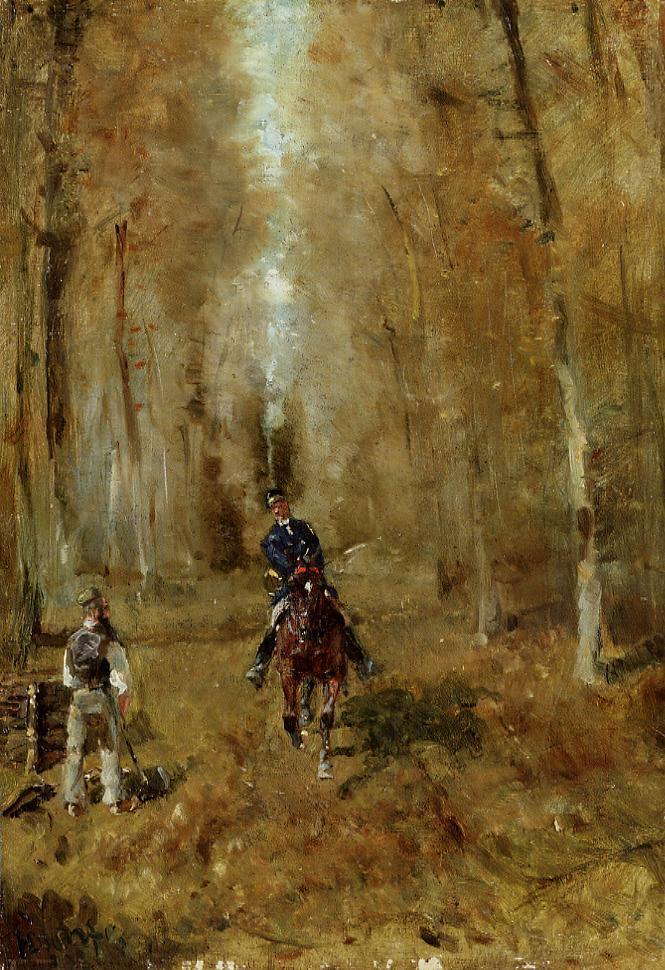In this detailed painting, set predominantly in warm earthy tones of brown and beige, a commanding figure in a striking blue police or military uniform rides a dark red horse straight towards the viewer. The horse, adorned with a distinctive white star on its forehead, is depicted with one leg bent backward, mid-stride. The rider's blue hat and uniform contrast boldly against the subdued, impressionistic backdrop of the woods.

To the left of the rider, standing on the brown forest floor, is another man. Dressed in a brown vest over a white shirt, gray pants, and a gray or green hat, this figure appears to be a farmer or lumberjack. He holds a rod or axe by his side, suggesting his occupation and underlining the setting’s rustic nature.

The forest scene is painted with a mix of gray and brown, with skinny tree trunks, perhaps withering under the autumn or early winter air. The sparse vegetation hints at a pathway cutting through the trees. A sliver of sky pierces the dense canopy, casting a blue light that illuminates the central figures amidst the sprawling shadows of the man and his horse. The painting cleverly balances the stark details of the central characters with the oblique, almost abstract depiction of their natural surroundings.